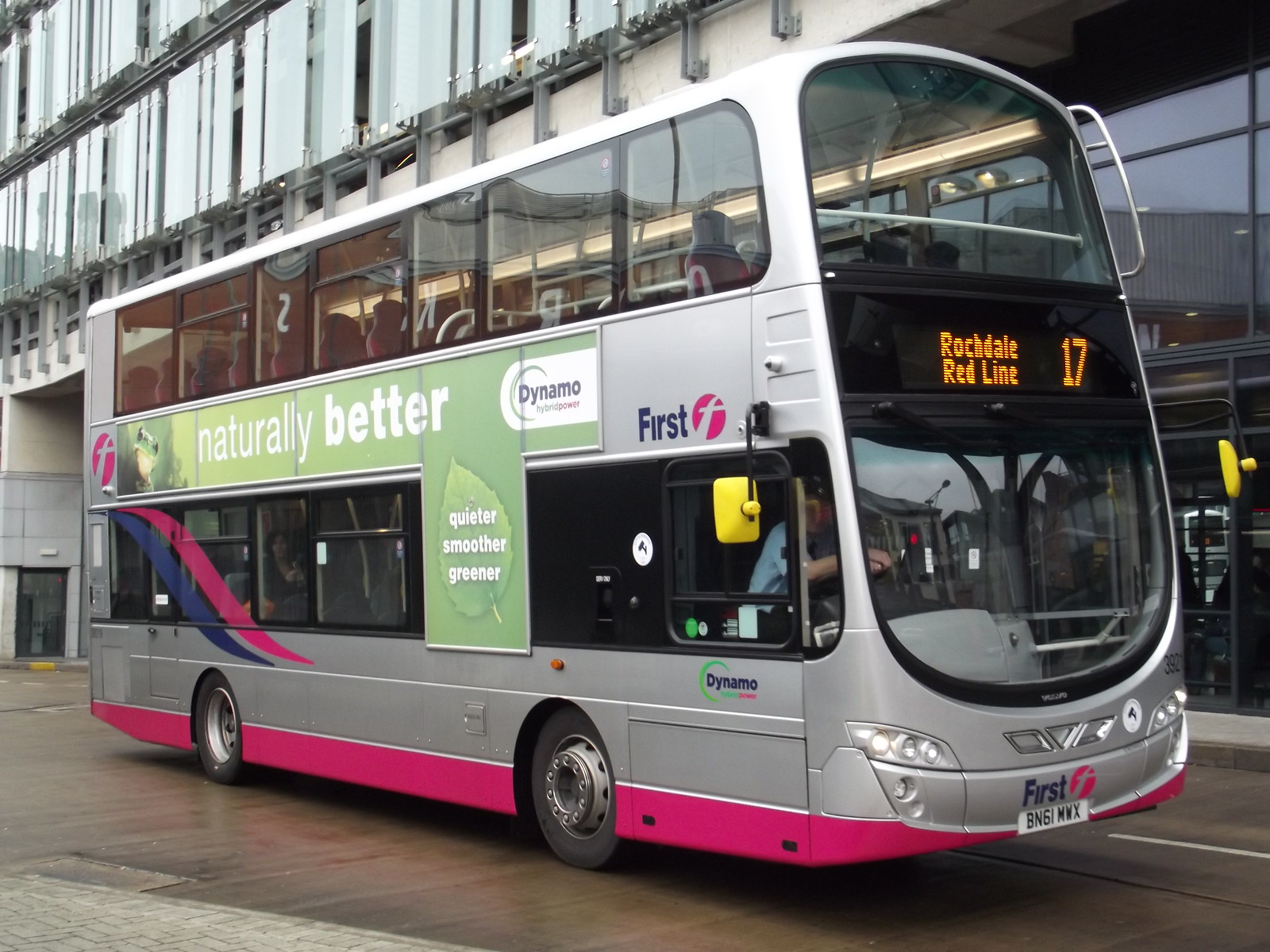This photograph, taken outside, features a vibrant double-decker bus as its main subject. The bus is predominantly gray with decorative elements, including a pink trim at the bottom and a swath of pink and blue towards the back. The sides of the bus are adorned with a green banner that reads, "Naturally Better, Quieter, Smoother, Greener" in white font. The bus prominently displays the route "Rockdale Redline 17" in orange on a black digital screen at the front, beneath which "First" is written in black with a pink circle containing an 'F' in negative space. The upper and lower levels of the bus are separated by a silver strip, also inscribed with the word "First." Passengers can be vaguely seen on the lower level, including a driver in a blue short-sleeve shirt and a passenger at the back. The backdrop consists of a modern building characterized by its numerous glass windows, metal, and concrete, with a clear view of the road pavement below. The picture's color palette includes various shades of gray, pink, blue, green, yellow, and orange, along with accents of clear, yellow, black, and silver.